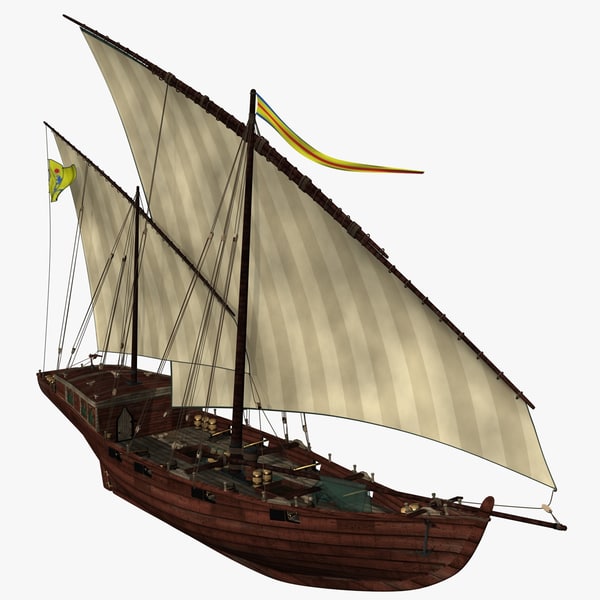The image depicts a computer-generated model of a brown wooden sailing ship reminiscent of a Viking vessel. The ship is positioned against a completely white background and is angled slightly towards the viewer, with the bow to the right and the stern to the left. The ship features two cream-colored, striped sails set bow to stern, one larger than the other, and both are angled with a high point on the left and a low point on the right. The larger sail is attached to a taller mast at the center of the ship, while the smaller sail is attached to a shorter mast on the left side. The ship’s deck includes yellow barrels and potentially green details inside. The ship also has an anchor at the bow and what appears to be a captain’s quarters at the aft. Additionally, there are two yellow flags: a long, thin one and a smaller banner-like one, both affixed to the top and top left of the masts. The exterior of the ship appears stained, enhancing its wooden appearance, and ropes can be seen attaching the sails.